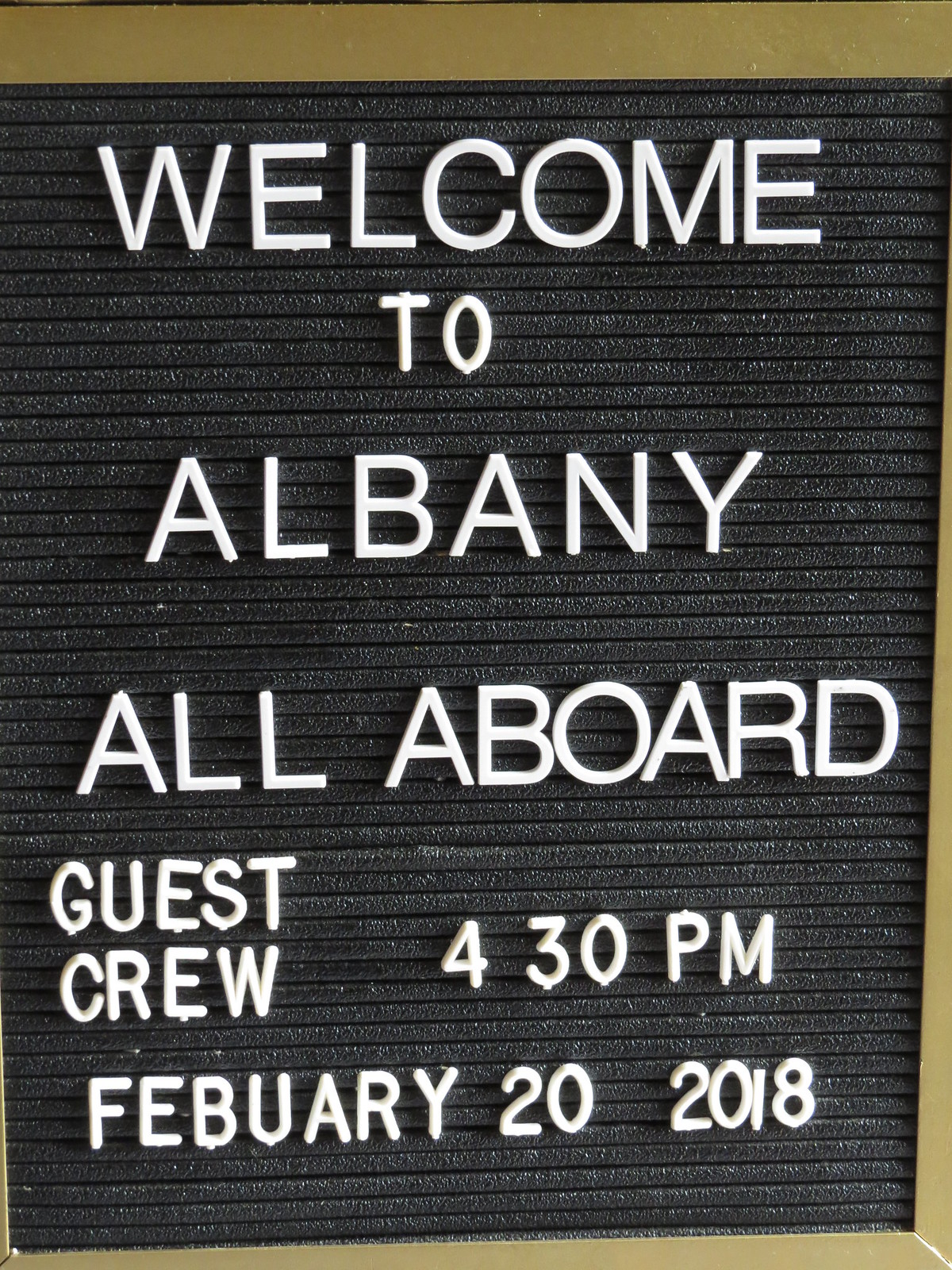The image depicts a photograph of a sign with a dark gray, textured background and horizontally ridged lines, allowing for customizable lettering. The sign, framed in gold that is visible on the top, bottom, and partially on the right side, displays white text reading, "Welcome to Albany, All Aboard, Guest Crew, 4:30 p.m., February 20th, 2018." The letters appear to be affixed on top rather than written directly on the surface, suggesting a vintage, changeable letterboard often used for announcements in train stations. Notably, the gold frame is mostly cropped out on the left side of the photograph. Despite its old-fashioned feel, the sign's date indicates it was still in use in recent years, making it a nostalgic touch in a modern era dominated by digital displays.